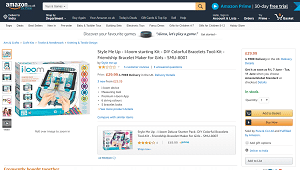The top of this image features a black banner with "Amazon.com" in white text. Below this banner, there are subtle accents of yellow and blue. Beneath that, a white search box is present, flanked by a small blue circle with a white arrow pointing to the right, labeled "Amazon Prime" in blue. This section also mentions either a "90-day" or "30-day" offer.

The primary focus is a main white box labeled "i-loom." To the left of this, there are seven smaller images vertically aligned. The main "i-loom" box is white with blue and gray accents, and is accompanied by several brightly colored items on the right in yellow, red, pink, purple, and blue. Information about these items is printed in purple, blue, and black text. On the right side, numbers are displayed in pink.

Towards the bottom right of the image, there are two small, light brown buttons with very small print. A gray box at the bottom includes a picture and a star rating of approximately three and a half stars. Finally, fine red print can be found at the very bottom of the image.